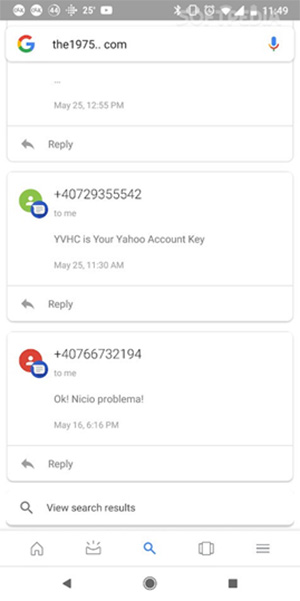This image is a detailed screenshot from a messaging app on an Android device. The status bar at the top of the screen shows a variety of icons, including notifications, signal strength, Wi-Fi connectivity, and battery level, which is nearly full. The current time displayed is 11:49 AM.

The main content of the screen features three separate message conversations, each housed in its own card for easy viewing and quick replies:

1. **First Conversation:**
   - **Sender**: (appears to be sourced from a search result on "the 1975...")
   - **Timestamp**: May 25th, 12:55 PM
   - **Message Content**: The preview shows an ellipsis (…). 
   - **Reply Option**: Available below the message.
   
2. **Second Conversation:**
   - **Sender**: Phone number 407-293-55542
   - **Timestamp**: May 25th, 11:30 AM
   - **Message Content**: "YVHC is your Yahoo account key."
   - **Reply Option**: Available below the message.
   
3. **Third Conversation:**
   - **Sender**: Phone number +407-667-32194
   - **Timestamp**: May 16th, 6:16 PM
   - **Message Content**: "Okay, Nikio, problema."
   - **Reply Option**: Available below the message.

At the bottom of the screen, various Android navigational icons are visible, enabling users to navigate through the app efficiently. Each message card includes essential information such as the sender's contact details, a time stamp, and a brief preview of the message content. This layout is designed to facilitate easy viewing and quick interaction with messages.